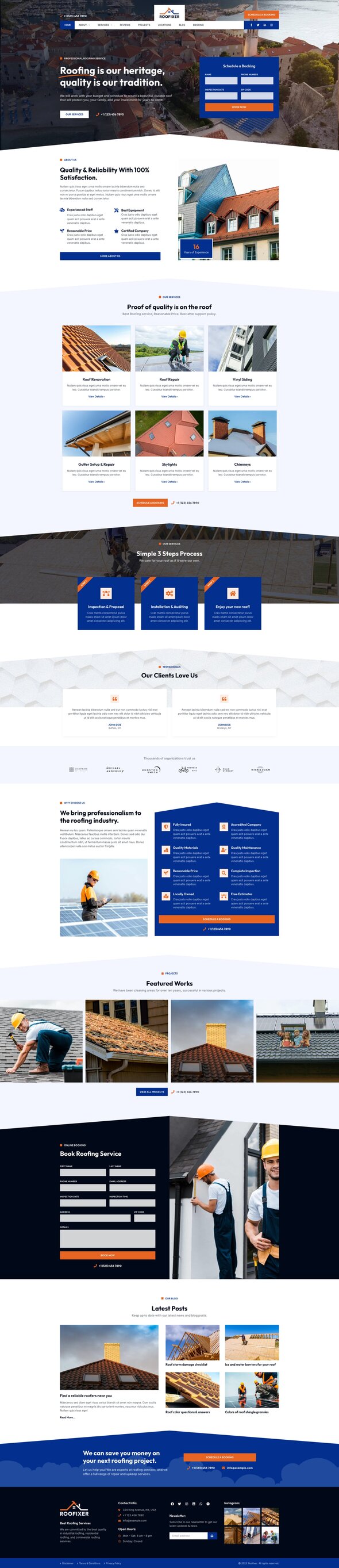A detailed screenshot of the website "Roof Fixer" features an elongated view encompassing multiple pages vertically. At the top, the "Home" page is highlighted within the navigation bar, which also includes sections such as About, Services, Reviews, Products, Locations, Blogs, and Booking. There are icons for social media links to Facebook, Twitter, and LinkedIn. A "Schedule Booking" button below allows users to input their information to book an appointment.

The watermark image in the header showcases a picturesque scene of closely-packed villas near the sea, hinting at an overseas location. Beneath this image, the taglines "Roofing is our Heritage, Quality is our Tradition" introduce the company's dedication to craftsmanship. Additional information describes the services offered, supported by a prominently displayed phone number.

A section titled "Our Services" encourages users to delve deeper by clicking a white button, indicating various offerings beyond roofing. "About Us" highlights the company's commitment to quality and reliability with 100% satisfaction, citing four key reasons: extensive experience (16 years), express equipment, certification, and reasonable pricing.

Following this, the website details their capabilities in roof restorations, roof repairs, vinyl siding, chimney repairs, skylights, and even satellite repair. A procedural outline explains their approach: inspect and propose solutions, install and audit, and finally, the customer enjoys their new roof.

A collage of images further down features clients, various types of roofs including clay drop-in roofs, and a man in a hard hat working on a roof. Also included are options to book roofing services and browse the latest blog posts. At the bottom, additional contact information is provided, including the company’s address, email, and hours of operation. More images are displayed alongside an option to subscribe to the company's newsletter.